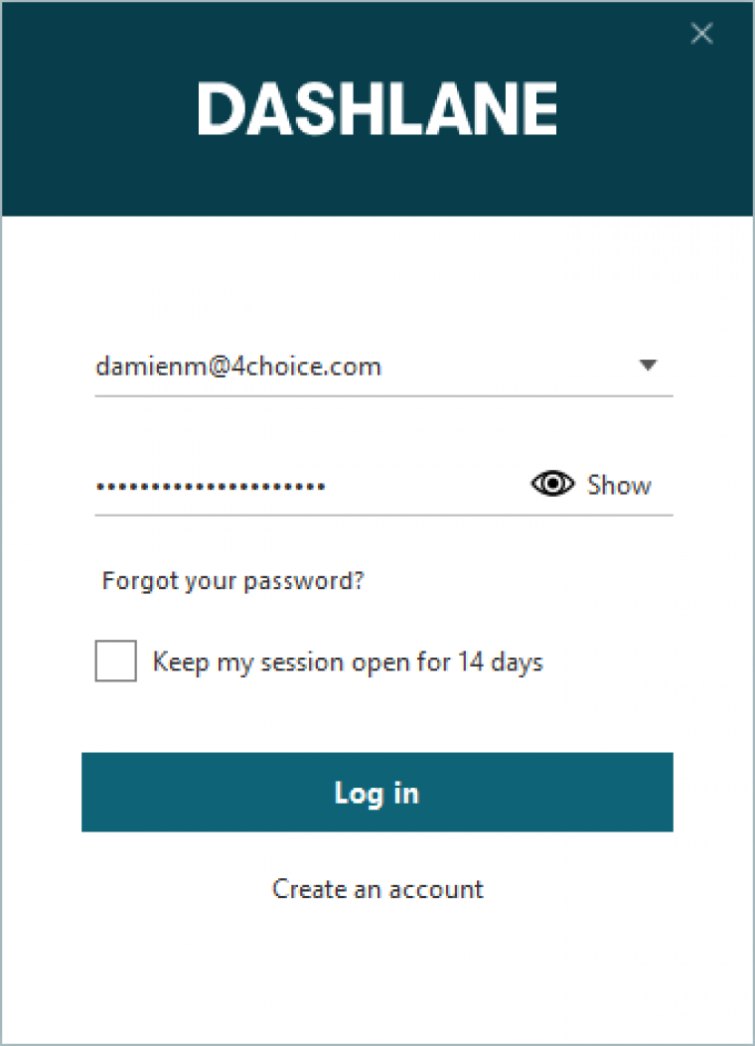A cropped screenshot of the Dashlane app interface features a blue banner at the top with the word "Dashlane" centered in bold white font. Beneath the banner, the background turns white, presenting the login section. A text box at the top displays a username or email address, followed by a drop-down box on the right side for switching logins. Below that, there's a password field filled with dots, indicating the password is hidden. Adjacent to this field on the right, an eye icon and the word "Show" in bold black font allow users to reveal the hidden password. Underneath the password field, the phrase "Forgot password?" appears in bold black letters to the left. Below this, a checkbox is present accompanied by the option "Keep my session open for 14 days," which remains unchecked. At the bottom, a large blue rectangle contains the word "Log in" centered in white font. Finally, beneath this button, the option to "Create an account" is displayed in smaller black letters.